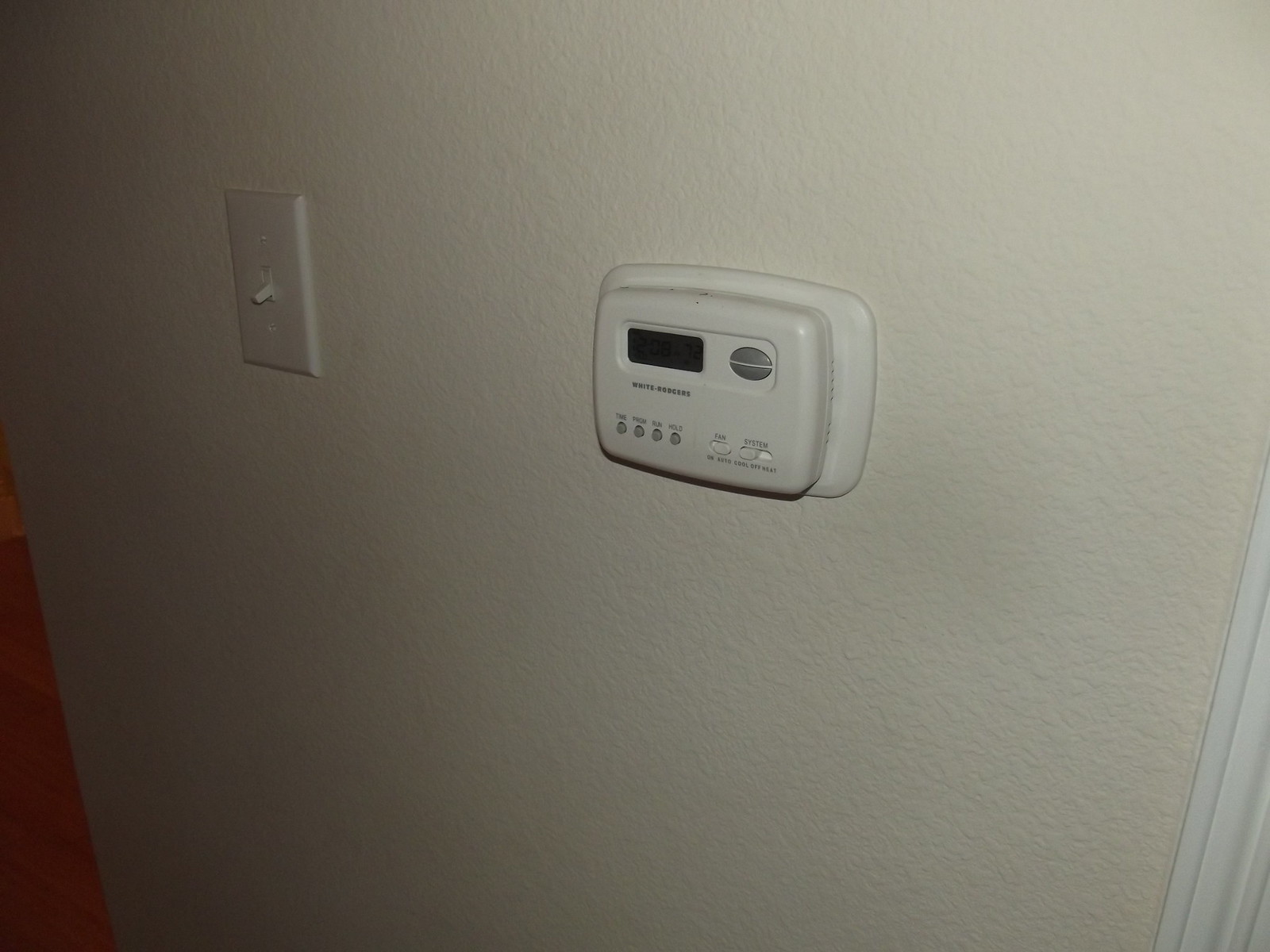This image shows a digital thermostat mounted on a textured cream-colored wall. The thermostat, which is positioned at the same height as a nearby light switch, suggests it's installed rather low on the wall. The device features a display screen without any visible digits, indicative of its digital nature. Below the screen are four small buttons. The thermostat includes a section for fan control with on and off settings. To the right of the screen, a gray semi-circular icon possibly indicates temperature readings. The thermostat is encased in a white base attached securely to the wall. There is white molding adjacent to the device, and a glimpse of hardwood flooring is visible at the bottom left corner, hinting at the room's overall design continuity in color.